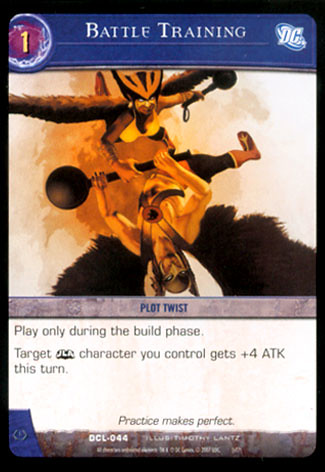The image is a detailed photograph of a rectangular playing card from a DC Comics trading card game. The card features a black border and a central rectangular section with beveled edges. At the very top is a horizontal blue stripe with the title "Battle Training" emblazoned in white. In the upper left corner, there is a white circle with a red background and a yellow number "1." The DC Comics logo is prominently displayed in the upper right corner.

Central to the card is an action-packed illustration of two superhero characters, Hawkman and Hawkwoman, engaging in an intense battle. Hawkman is depicted upside down in mid-air, clutching his signature weapon with a ball and chain, while Hawkwoman, with her black wings outstretched, is swooping down from above, ready to strike with her own weapon.

Below the illustration, a horizontal gray bar with blue text reads "Plot Twist." Underneath this bar, there is a white rectangle with black print that states, "Play only during the build phase. Target JLA character you control gets +4 ATK this turn. Practice makes perfect." The bottom of the card has additional text that is too small to read clearly. The card, overall, signifies a battle training scenario and is part of a card game involving strategic gameplay with recognizable DC Comics characters.